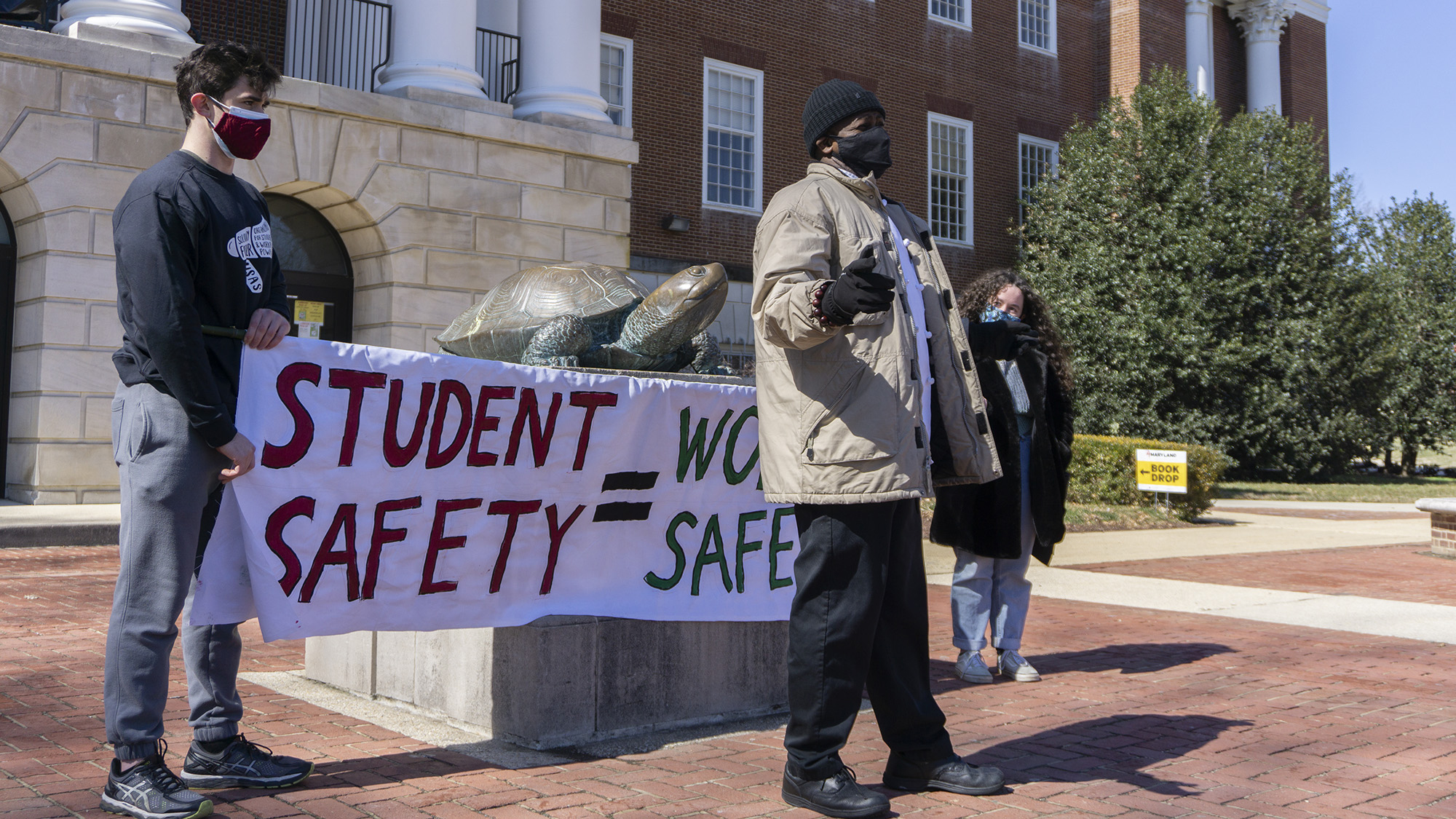This photograph captures a scene outside a college campus during the daytime, showcasing three people standing on brick ground in front of a large, red brick building adorned with white columns and arched doorways. Dominating the composition is a man positioned centrally, viewed from the side. He is attired in a tan jacket, black jeans, black shoes, and a black hat, and he is wearing a mask, indicative of the COVID-19 era. His arms are outstretched as if he is addressing a crowd or giving a speech.

Behind him, a woman and another man are holding a prominent white banner. The sign reads "Student Safety Equals Work Safety" in a mixture of red, black, and green lettering, with the words "Student Safety" in red, the equal sign in black, and "Work Safety" in green. The scene is set against a backdrop featuring a brass turtle statue situated on a cement block, adding a distinctive element to the image. This statue and the surrounding trees contribute to the picturesque nature of the college campus environment.

The people in the photograph appear to be of European descent and are all wearing masks, reinforcing the timeframe as the pandemic period. The clear skies and daylight suggest a mild, likely pleasant day on campus, further emphasized by the presence of a small sign that reads "book job," implying proximity to the campus library.